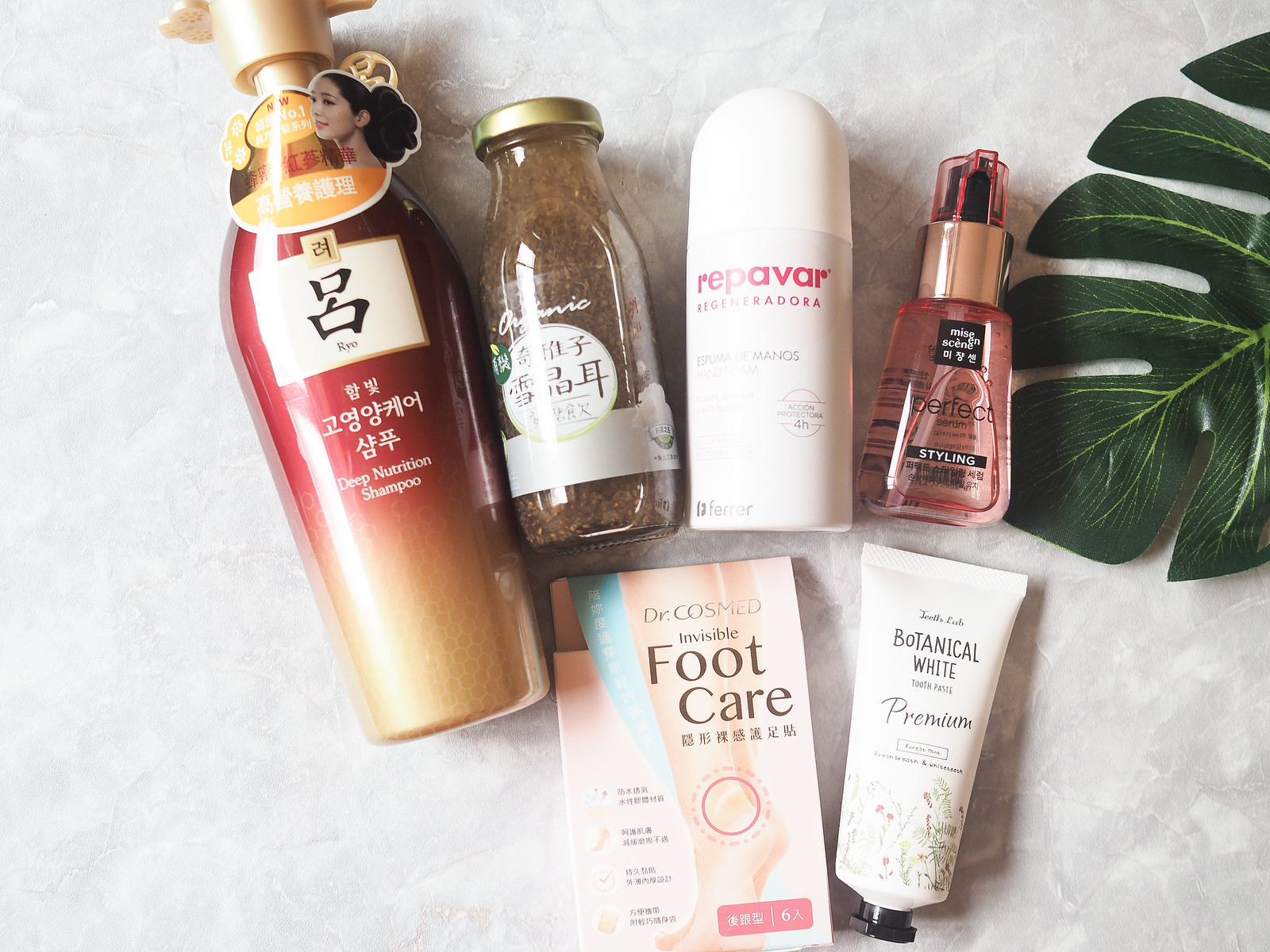This top-down photograph beautifully captures six meticulously arranged personal care items placed on a marbled dove gray background. In the upper right-hand corner of the image, part of a lush, deep green monstera leaf graces the frame, its iconic split leaves adding a touch of organic elegance.

The six bottles are arranged with four in the top row and two in the bottom row. Starting from the bottom row, on the left, there's a peach-colored box labeled "Dr. Kozmed Invisible Foot Care" featuring detailed instructions and various symbols in chocolate brown and black fonts. To its right, there's an ivory tube with a black screw cap adorned with botanical illustrations of flowers, leaves, and stems, marked "Botanical White Premium."

Moving to the top row, from left to right, the first item is a luxurious glass bottle of shampoo, transitioning from a gold top to a metallic orange hue, with a sophisticated gold screw cap. It bears both Asian characters and the English text "Deep Nutrition Shampoo." Beside it is a jar that resembles a condiment container, with a gold screw cap and filled with a substance that looks akin to chutney, labeled "Organic." Next, there is a white plastic container with a cone-style twist top, branded "Repavar" in elegant pink, lowercase font. Lastly, there is a glass bottle containing a light pink styling gel, equipped with a push pump for convenient dispensing.

The thoughtful arrangement and detailed presentation make this a visually appealing image, showcasing the diverse range of personal care products against a stylish, modern background.